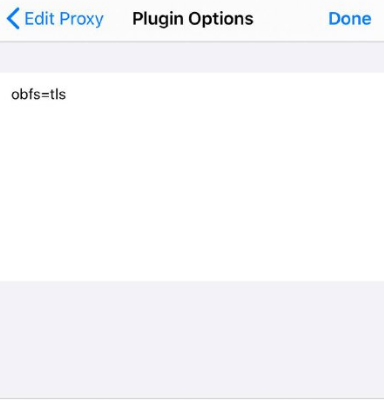The image features a predominantly monochromatic design with distinct sections of varying shades of gray and white. The top inch of the image is an almost white, light gray color. In the top left corner, a prominent, bold blue greater-than sign points to the right. To the immediate right of this symbol, in the same blue color, are the words "Edit Proxy" with the letters "E" and "P" in uppercase.

Centrally positioned and bolded in black are the words "Plugin Options," with "P" and "O" capitalized. On the far right side of this section are the words "Done," also bolded and in blue, with the letter "D" capitalized.

Below this is an inch-high section of a slightly darker gray, which lacks any content. A subtly darker horizontal line separates this gray section from the white area that extends downward to about two inches from the bottom of the image. In the top left corner of this white section, in smaller, bold black letters, are the characters "OBFFS", followed by an equals sign and "TLS". 

The remainder of this white section is empty until approximately two inches from the bottom, where it transitions into a lighter blue-gray area. This bottom section, which continues to be empty, is capped off with a slightly darker horizontal line running across the entire width of the image.